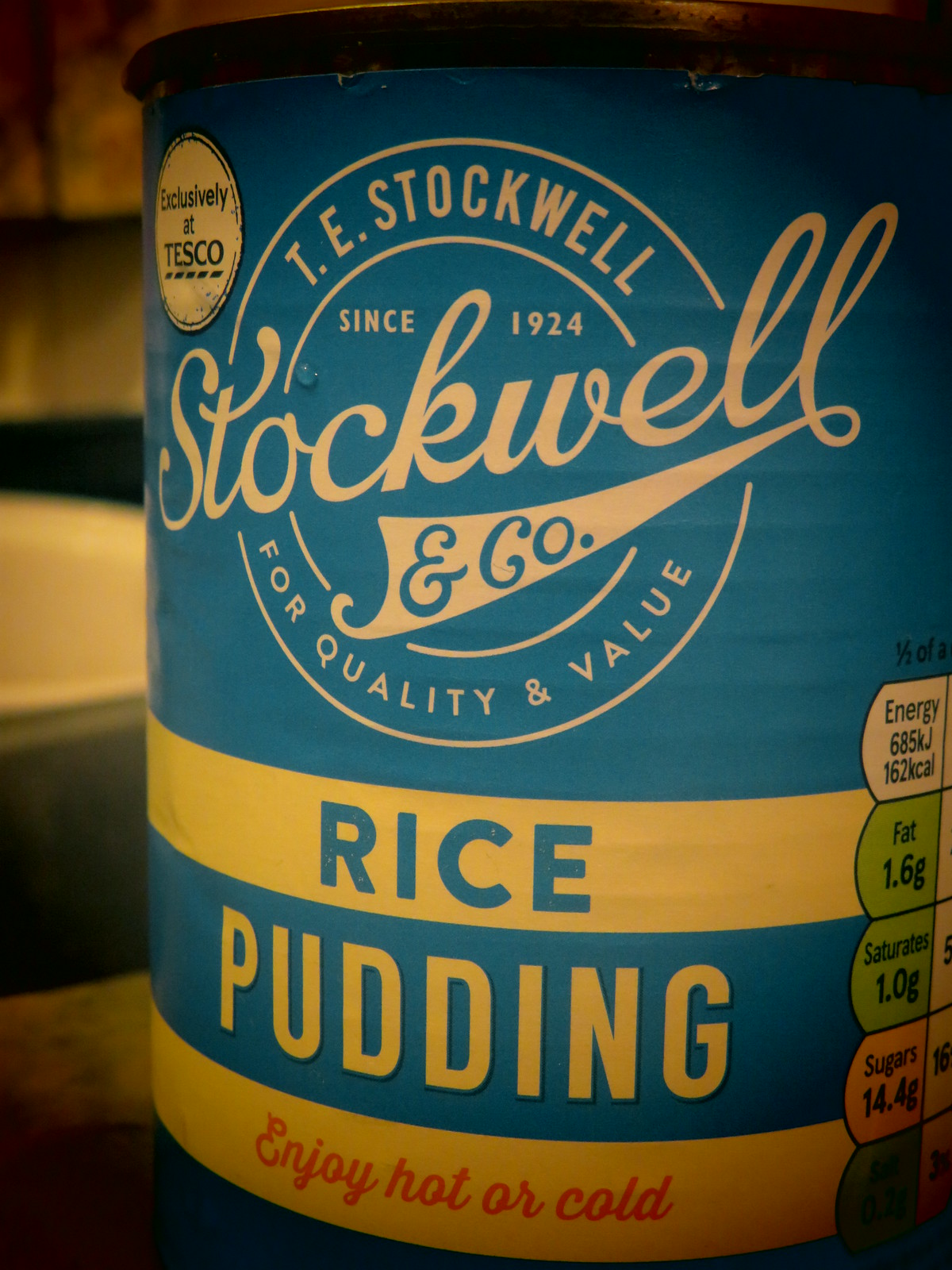The image presents a close-up of a metal can, prominently featuring its detailed label designed with visual clarity and vintage appeal. The upper half of the label is light blue, adorned with a white circular logo framed by two concentric white lines. Inside this circular logo, the text reads "T. E. Stockwell," and the bottom curve contains the phrase "For quality and value," with "Stockwell and Company since 1924" elegantly scripted through the center.

Beneath the logo, the label displays three horizontal stripes: the first and third are yellow, and the middle is blue. The top yellow stripe has the word "Rice" in blue text, while the blue stripe below it declares "Pudding" in bold yellow text. The bottom yellow stripe encourages the consumer with "Enjoy hot or cold" written in red cursive.

To the right-hand side of the label, nutritional information is listed with precise measurements: "Fat 1.6g, Saturates 1.0g, Sugars 14.4g." Additionally, the can mentions energy content, specified as "685 KJ / 162 kcal."

This can of rice pudding, marketed as exclusive to Texco, embraces traditional branding elements and clear nutritional details, making it both nostalgic and informative.